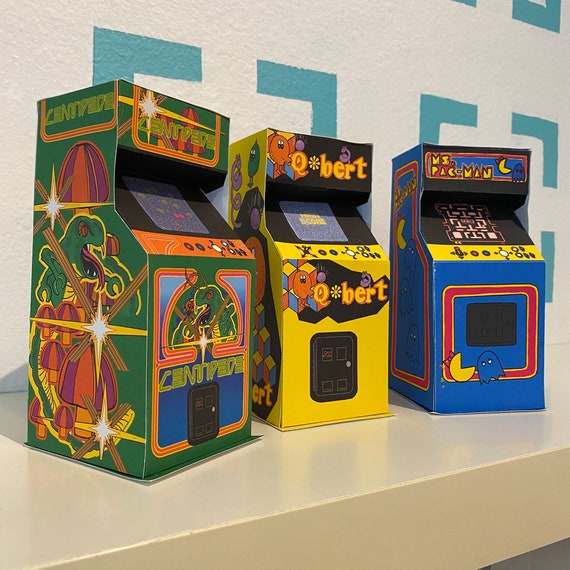The image features three classic arcade cabinets lined up in a row against a white wall adorned with green square symbols. The cabinets, replicas from the late 80s or 90s, are placed on a white floor and appear slightly angled, creating a dynamic display.

On the far left is the iconic "Centipede" cabinet. The main color is green, with orange and yellow trim. It features a detailed, eerie depiction of a giant centipede and mushrooms on both the side and front. The game's title, "Centipede," is prominently displayed in three locations on the cabinet.

In the center is the "Q-Bert" cabinet, predominantly yellow with black trim. The cabinet showcases the quirky, orange, elephant-like character Q-Bert on both the upper section and lower front. 

The rightmost cabinet is for "Ms. Pac-Man," distinguished by its blue color with red trim. Ms. Pac-Man, depicted in yellow text with red accents, appears on the top of the cabinet. The front lower half features her about to munch on a blue ghost, encircled by a red ring.

Together, these cabinets capture the nostalgia and vibrant artwork characteristic of classic arcade games, each adorned with colorful and engaging illustrations of their respective characters and themes.